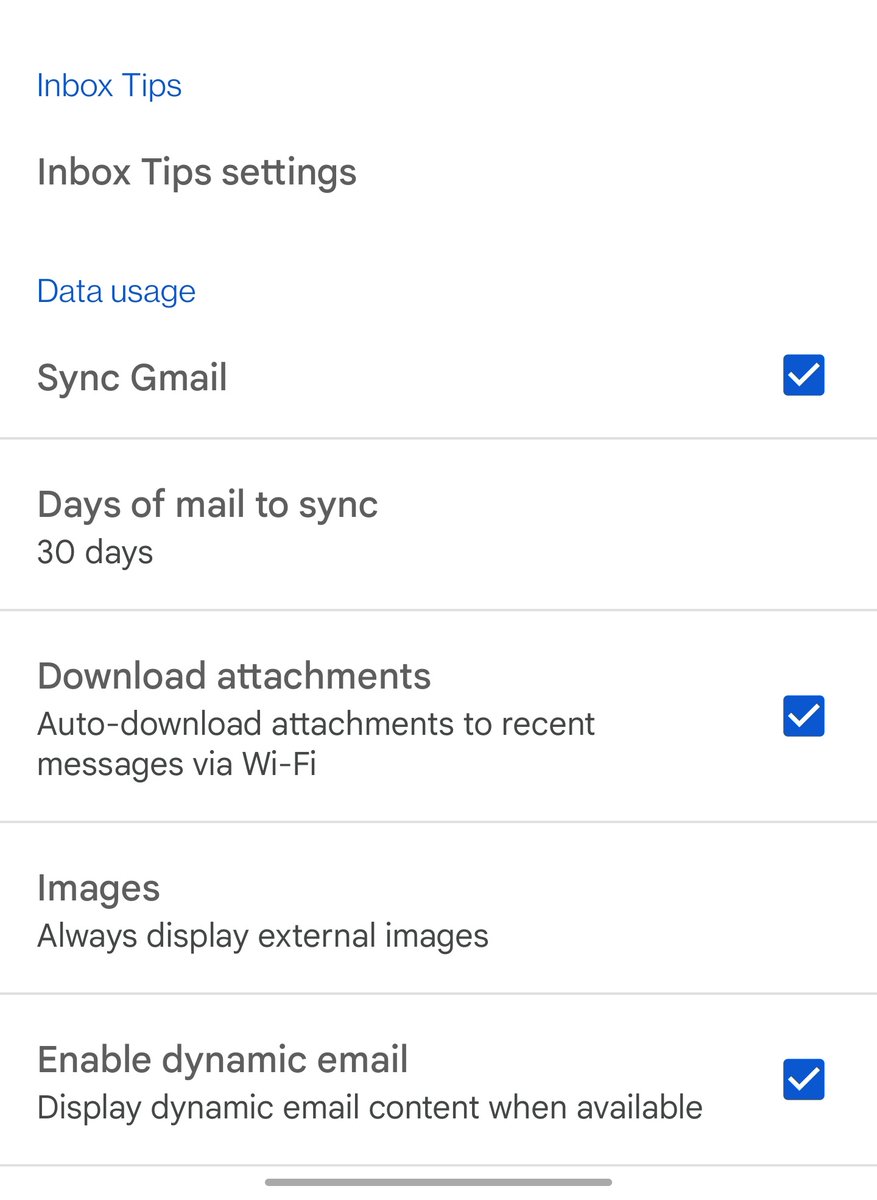The image is a screenshot of a settings page from a mobile app or website, specifically focusing on email account settings. The background is primarily white. At the top of the page, in small blue text, the title "Inbox Tips" is displayed. Below this, in slightly larger dark grey text, it reads "Inbox Tip Settings." Further down, "Data Usage" is written again in small blue text.

The settings are segmented into different sections, each separated by a light grey line, and written in dark grey text. The first section is labeled "Sync Gmail," with a blue checkbox to the right indicating it is enabled. Below this, "Days of Mail to Sync" is set to "30 days."

The next line reads "Download Attachments," followed by a description: "Auto Download Attachments to Recent Messages via Wi-Fi." Next to this, a blue checkbox shows this feature is enabled.

Following that, the section labeled "Images" specifies that it will "Always Display External Images."

The final section, "Enable Dynamic Email," states that it will "Display Dynamic Email Content when Available." Each of these options has a corresponding blue checkbox on the right, all of which are shown as being checked.